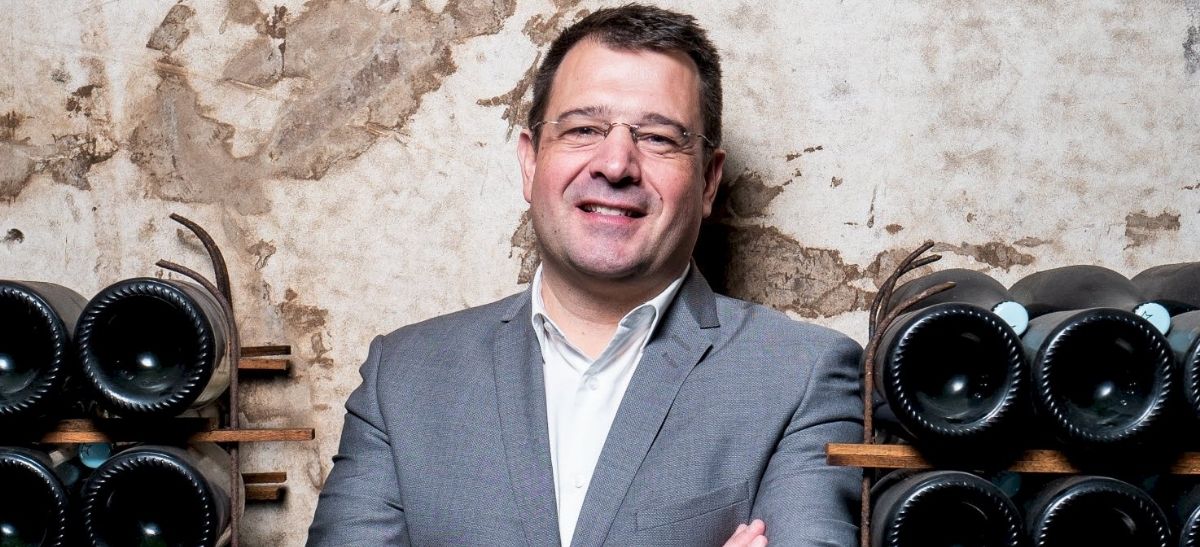A photograph captures a Caucasian man in his early 50s, his light-colored skin and short brown hair adding to his distinguished yet approachable look. He wears thin, rimless glasses and a charcoal gray suit paired with a white shirt. His face shows a bit of a five o'clock shadow. The man stands against an old, peeling light beige wall, giving the scene a sense of age and wear. He's wedged between two wooden shelves filled with wine bottles, their dark bottoms facing outward, suggesting they are red wines. The scene is further framed by the arm-crossed stance of the man, though the image crops out his arms below the elbows. The overall impression is one of quiet elegance amidst a rustic, slightly decrepit setting.